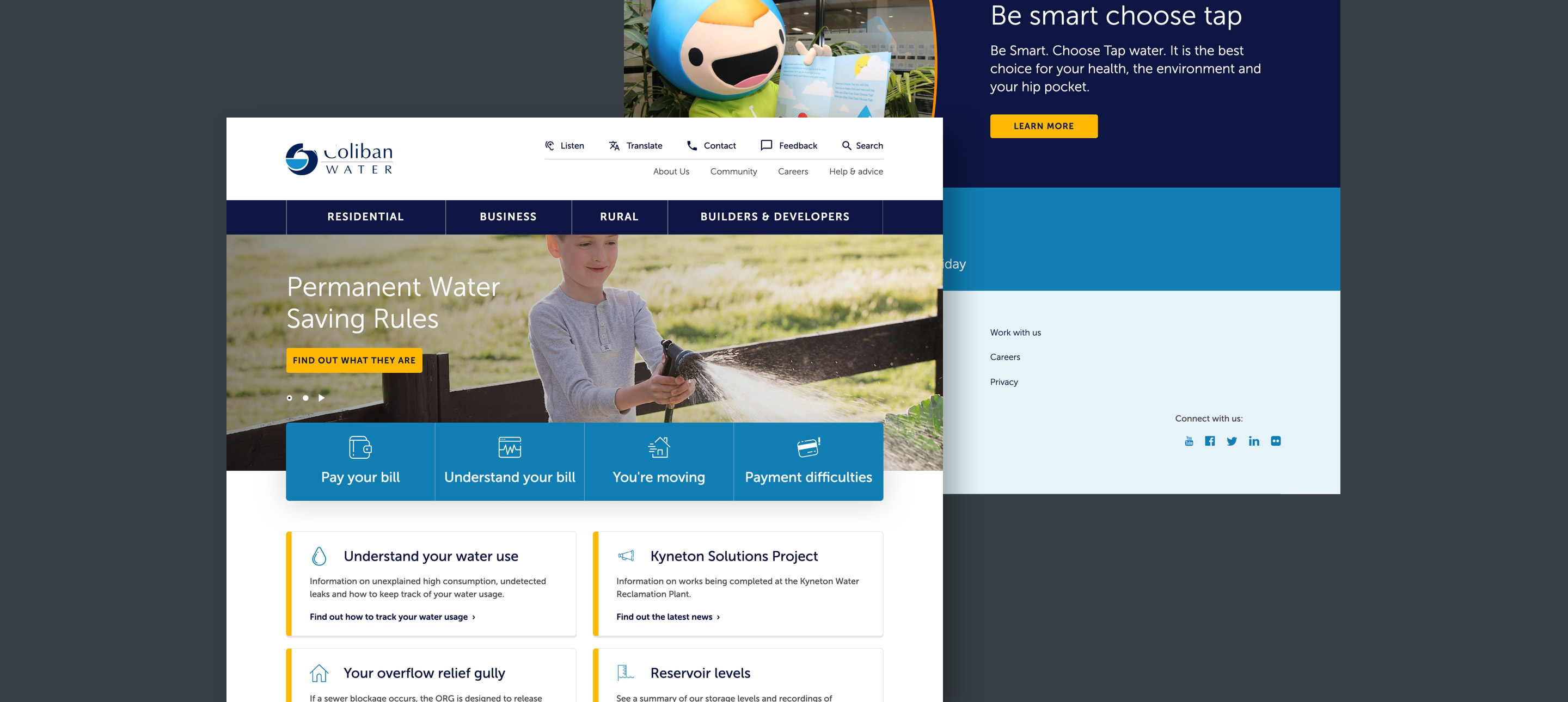This photograph captures two juxtaposed website interfaces. On the left side, the website is titled "Koloban Water." The page predominantly features a clean white background with blue text. Directly beneath the Koloban Water logo is a dark blue navigation bar with white text featuring links for "Residential," "Business," "Rural Builders," and "Developers." Below this navigation bar is an image of a boy playing with a hose, spraying water outdoors. Adjacent to this, there is a message about "Permanent Water Saving Rules" presented in black text on a yellow bar, with a call to action that reads "Find Out What They Are."

Further down, another set of links is displayed, labeled "Pay Your Bill," "Understand Your Bill," "You're Moving," and "Payment Difficulties." Towards the bottom of the website, additional links are available, including "Understand Your Water Use," "Chitin Solutions Project," "Your Overflow Relief Gully," and "Reservoir Levels."

On the right side of the photo, an illustrated character resembling a boy in a blue hat is prominently displayed. The accompanying text encourages viewers to "Be Smart, Choose Tap," emphasizing the benefits with the statement "Be Smart, Choose Tap Water. It's the best choice for your health, the environment, and your hip pocket." A yellow bar further invites users to "Learn More."